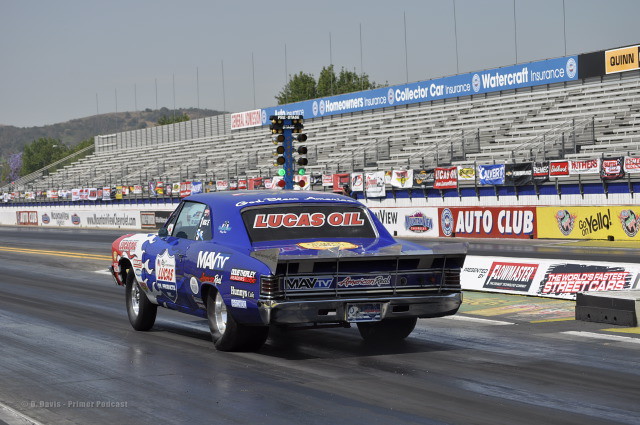In this detailed image, we see a blue race car prominently positioned on a black racetrack, likely a drag strip, given the context. The car is adorned with numerous logos and symbols, the most striking of which is "LUCAS OIL" displayed in bold red letters on the front, top, back, windows, bumper, and rear windshield. "MAV TV" is prominently featured on the side along with various other logos. The racetrack is lined with a long protective wall covered with advertisements and company logos similar to those on the car. The empty white bleachers above suggest a practice run, with more company banners displaying advertisements such as "homeowners insurance," "collector car insurance," and "watercraft insurance." Farther along, another banner reads "general custom." The image is set against a backdrop of blue skies, with mountains and trees in the distance, giving a scenic yet professional racing environment. The car is captured moving from left to right, creating a dynamic sense of speed and motion.